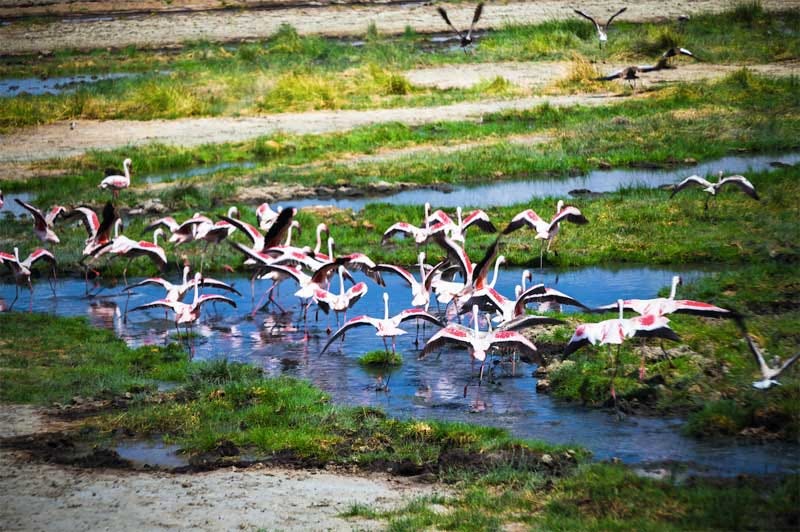This vibrant and lively photograph captures a dynamic scene in a marshy wetland area bustling with the activity of at least forty flamingos, exuding their characteristic pink tint with white plumage and black-tipped wings. The birds are engaged in playful behavior and appear animated or distressed, dashing across shallow, sparkling waters that splash under their long legs. Strips of vivid green grass intersperse the scene, creating a patchwork with the shallow, clear blue water that reflects the bright sunlight. Amongst the flamingos, which dominate the foreground in their display, some seagulls can be observed flying around, possibly in search of food or driven by the commotion of the flamingos. The landscape suggests a locale outside America, showcasing a lush, expansive flat land with sandy patches and a road-like strip in the background, contributing to an overall picturesque and immersive visual experience.